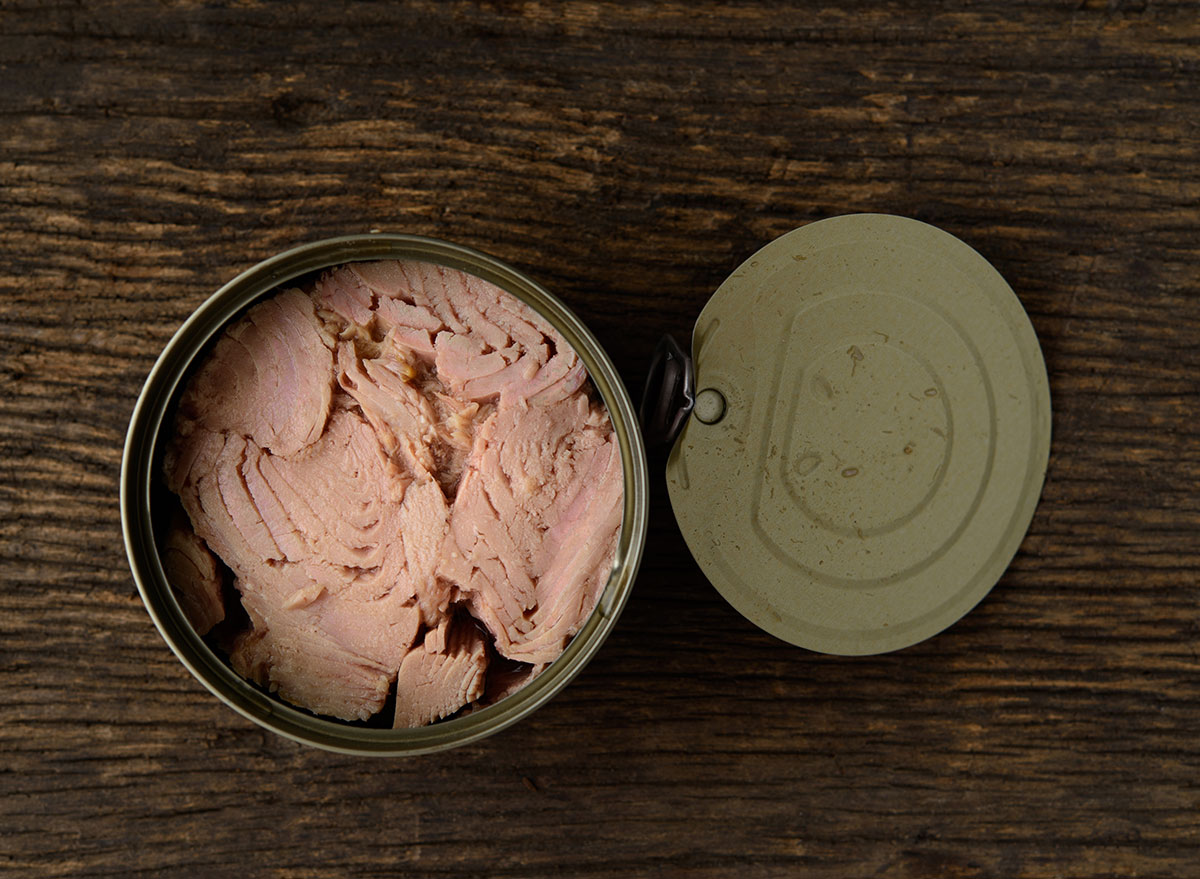The image features a can of pinkish meat, possibly tuna or another type of processed meat, opened and placed on a dark, grainy wooden table. The wooden surface is stained a deep brown, highlighting its textured grain lines. The can, viewed from above, is centered slightly to the left. The bronze-colored rim and the inside of the open can contrast with the dense, chopped meat packed tightly within. The lid, displaying its bronzy gold underside and silver pull tab, rests at an angle next to the can on the right. The detailed perspective showcases the compressed slices of meat, suggesting it could be used in a recipe or a sandwich, and hints that it might even be suitable as pet food.